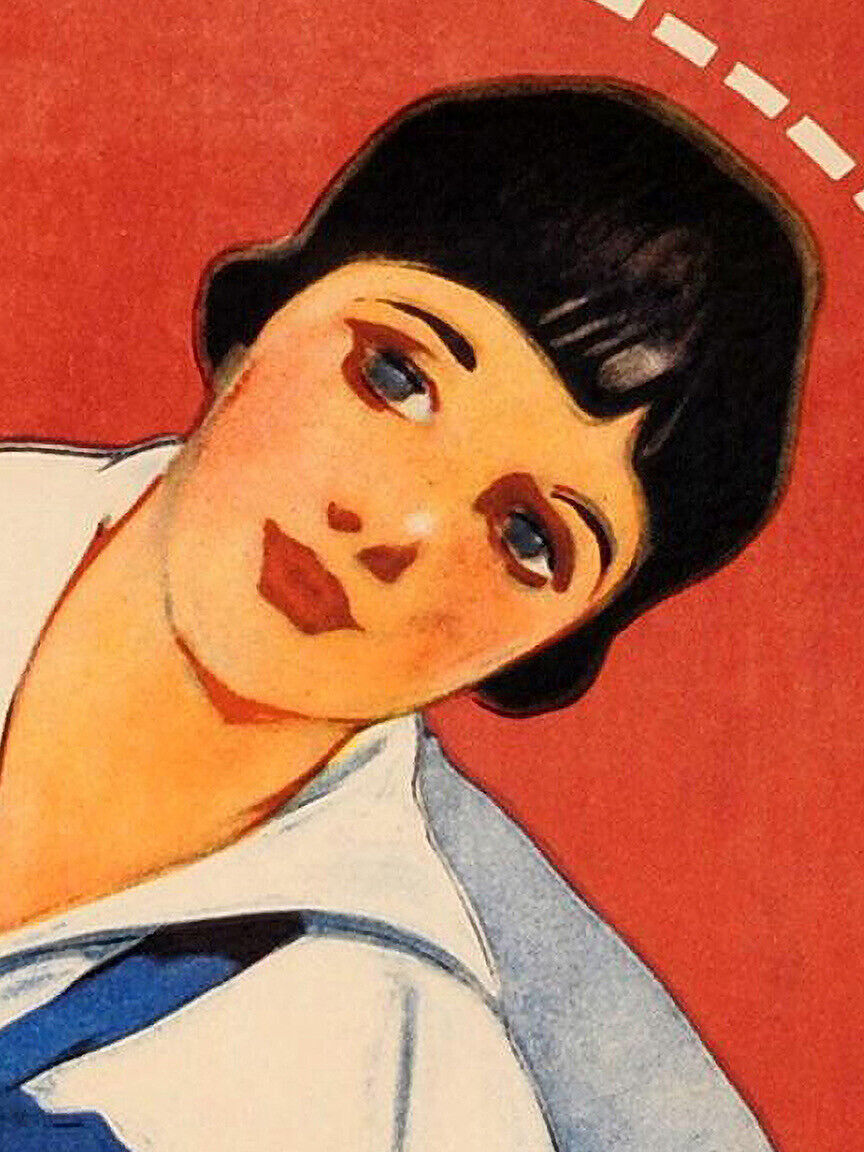The image depicts a stylized, vintage painting reminiscent of an old World War II poster. The artwork, oriented vertically, features a woman with black, page boy cut hair and dark eyebrows, wearing a white sailor's outfit accented with blue ribbon-like details. Her skin is light, and she has distinct red, painted lips with blue or grayish-blue eyes. The woman's head and body are tilted to the right against a reddish background, which is punctuated by dotted white lines running across the upper right corner, resembling a roadway's markings. Below and to the right of her head, a pattern of white and blue can be seen, which might represent the edge of a sofa. The entire scene evokes a nostalgic, historical ambiance, capturing the essence of mid-20th-century art styles and themes.